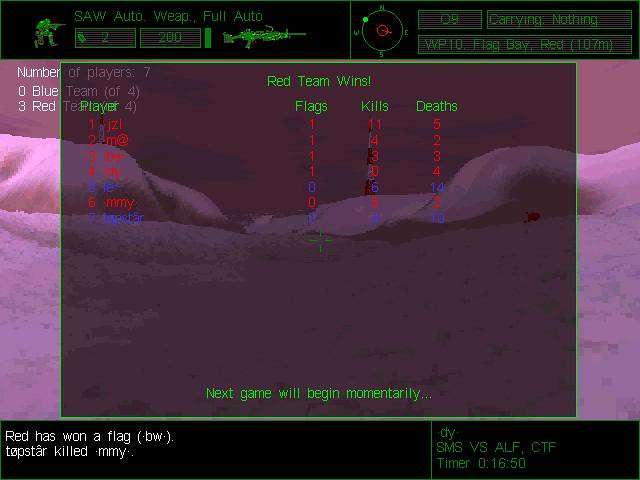The image is a screen grab from a video game showing the end of a match. The top of the screen features a black band with a crouched figure holding a gun, labeled "SAW Auto," "Full Auto," and other details including "W Auto," "38p," and "200." To the left, there are coordinates and various game-related stats such as "09," "Carrying Nothing," "WP10," "Flag Bay," "Red," and "107M." Below this, there's a bright green icon of a gun and the figure.

At the bottom of the screen, another black band displays a message in white text: "Red Has Won a Flag" and "Top Star Killed MMY." The central area is a mix of dark and light purple hues. A semi-transparent rectangle dominates the middle, stating "Red Team Wins" in bright green, along with categories for "Player," "Flags," "Kills," and "Deaths." Another message reads, "Next Game Will Begin Momentarily" followed by three dots. Additional information indicates the game's score: "Blue Team: 0" and "Red Team: 3."

Overall, the screen indicates that the match is over, with the red team emerging victorious, and a new game is about to start soon.